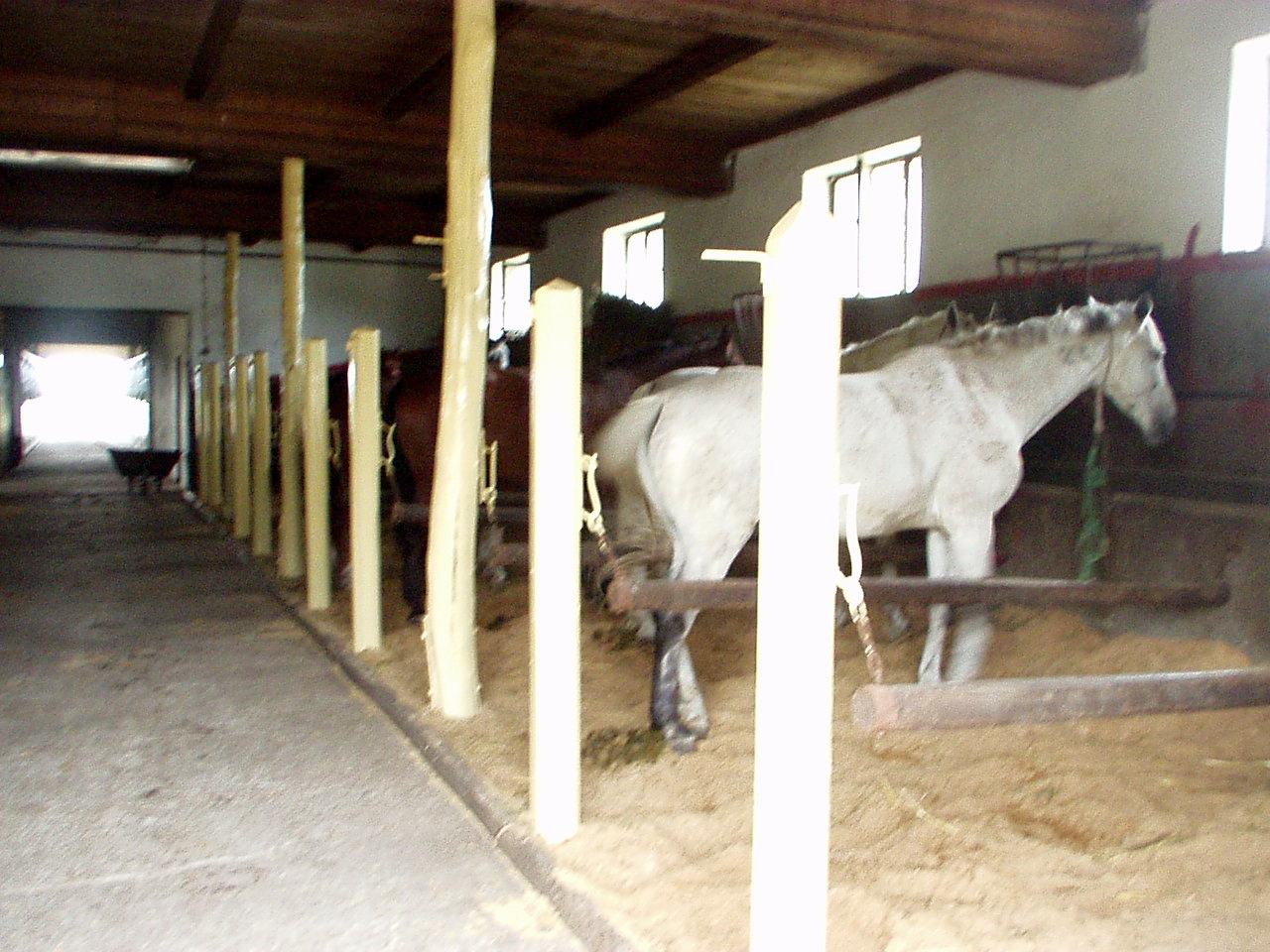This photograph captures the inside of a barn or outdoor stall area, with a wooden roof and exposed dark brown beams. The structure features a gray concrete walkway running through its entire length, leading to a square door at the back where light shines through. The right-hand side of the image is lined with horse stalls, separated by light brown wooden posts. The ground of the stalls appears to be a mixture of dirt, sand, and hay. 

In the foreground, a white horse with darker colored ears, feet, and mouth, is tethered to the wall of its stall by a green rope. The horse stands sideways, with its head pointed to the right and tail to the left, revealing a partial view of other horses in the stall area. Behind this horse, glimpses of brown and other indistinct colored horses can be seen. The barn's walls include white sections, and windows are visible in front of the horses.